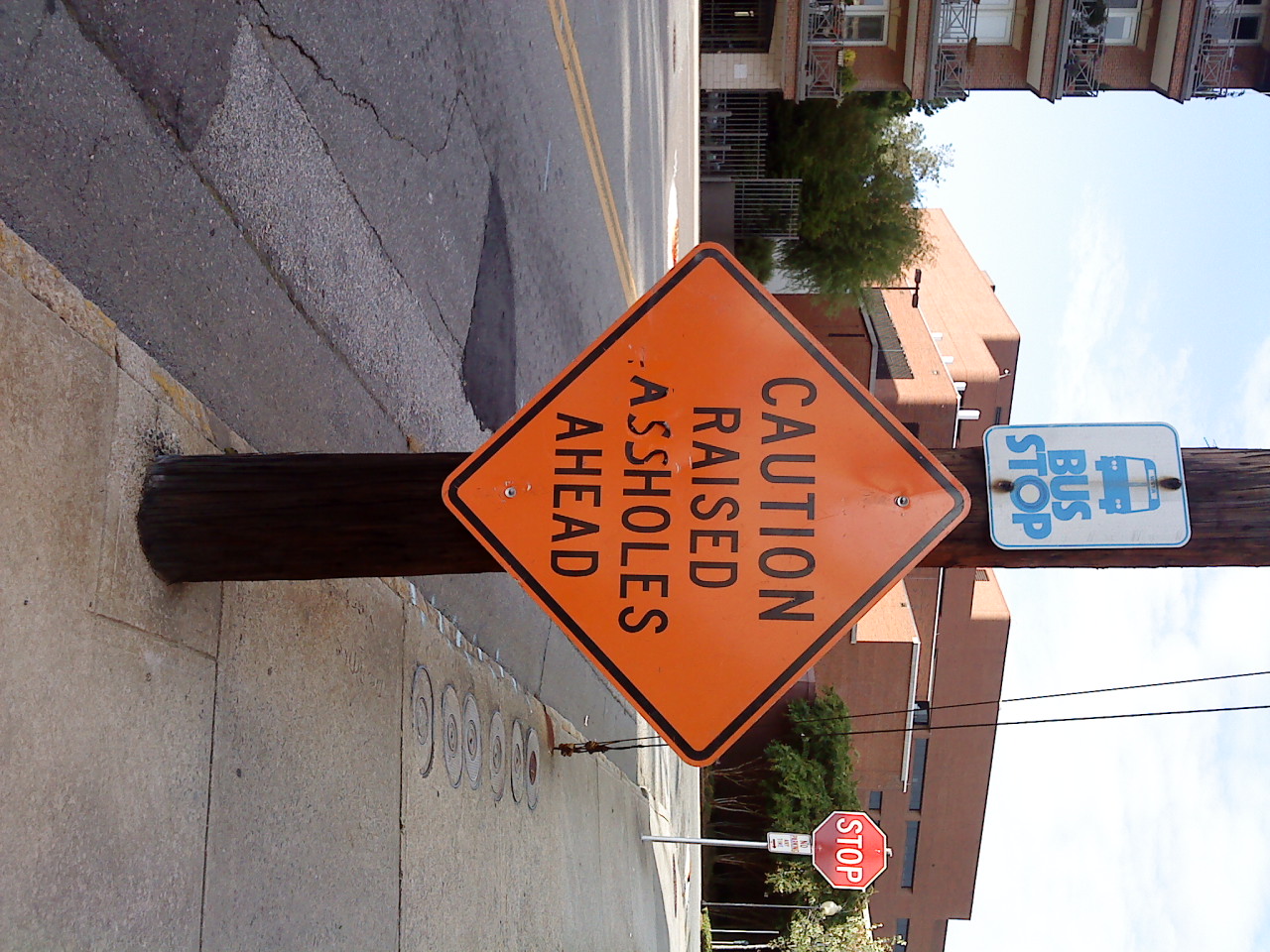The image shows a busy public street corner dominated by a large brown utility pole adorned with two signs. The upper sign is a white bus stop sign featuring a blue bus icon and the text "BUS STOP" in bold blue letters. Below it, an orange caution sign with black lettering has been humorously altered by graffiti to read "CAUTION RAISED A.S.S.H.O.L.E.S AHEAD," clearly not an official traffic sign. The background reveals a mid-rise red brick apartment building to the left, complete with balconies, and another multistory brick building that appears to have minimal natural light, suggesting it might be a different kind of facility. A cracked and patched asphalt street, marked by a double yellow center line, runs horizontally through the image. The concrete sidewalk runs parallel to the street, with a red stop sign visible at the far end of the block. The scene is bathed in sunlight, highlighting the details and textures of the urban setting.